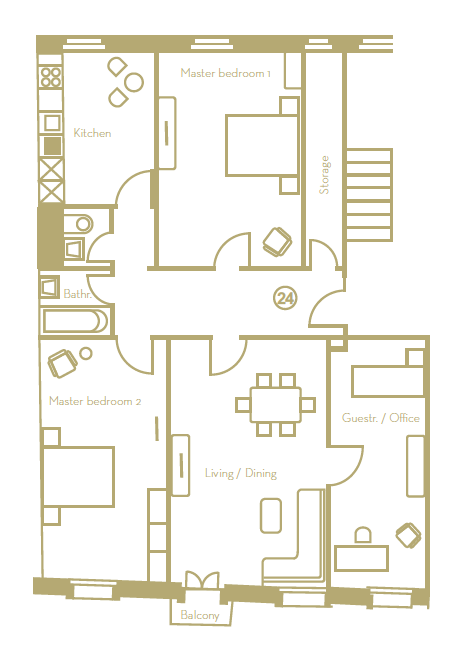This diagram provides a detailed overhead view of a house layout. The image is predominantly white, with labels in a light brown color for easy identification. 

Starting from the right-hand side on the bottom layer, the layout features a lengthy storage area. Adjacent to this storage area is a space designated as the master bedroom (#1). Directly behind the master bedroom is the kitchen, providing easy access to both areas. Next to the kitchen, there is a small space that appears to be a closet or a washroom. Proceeding down the hallway, a bathroom is positioned straight back.

In the front corner of the house is what is labeled as the master office room, leading into a large living room. Another master bedroom (#2) is also situated within this area. The diagram highlights a small front porch with a section delineated as a "little slat."

A notable feature in the diagram is a circle marked with the number "24" located in the center of the hallway, though its significance is unclear. Each room in the house is equipped with a single window to allow natural light in. The master bedroom (#1) and the living room share proximity to a bathroom, which is accessible from the hallway near the master bedroom.

This comprehensive overhead view offers a clear and concise depiction of the house's floor plan, ensuring all areas and features are easily understood.